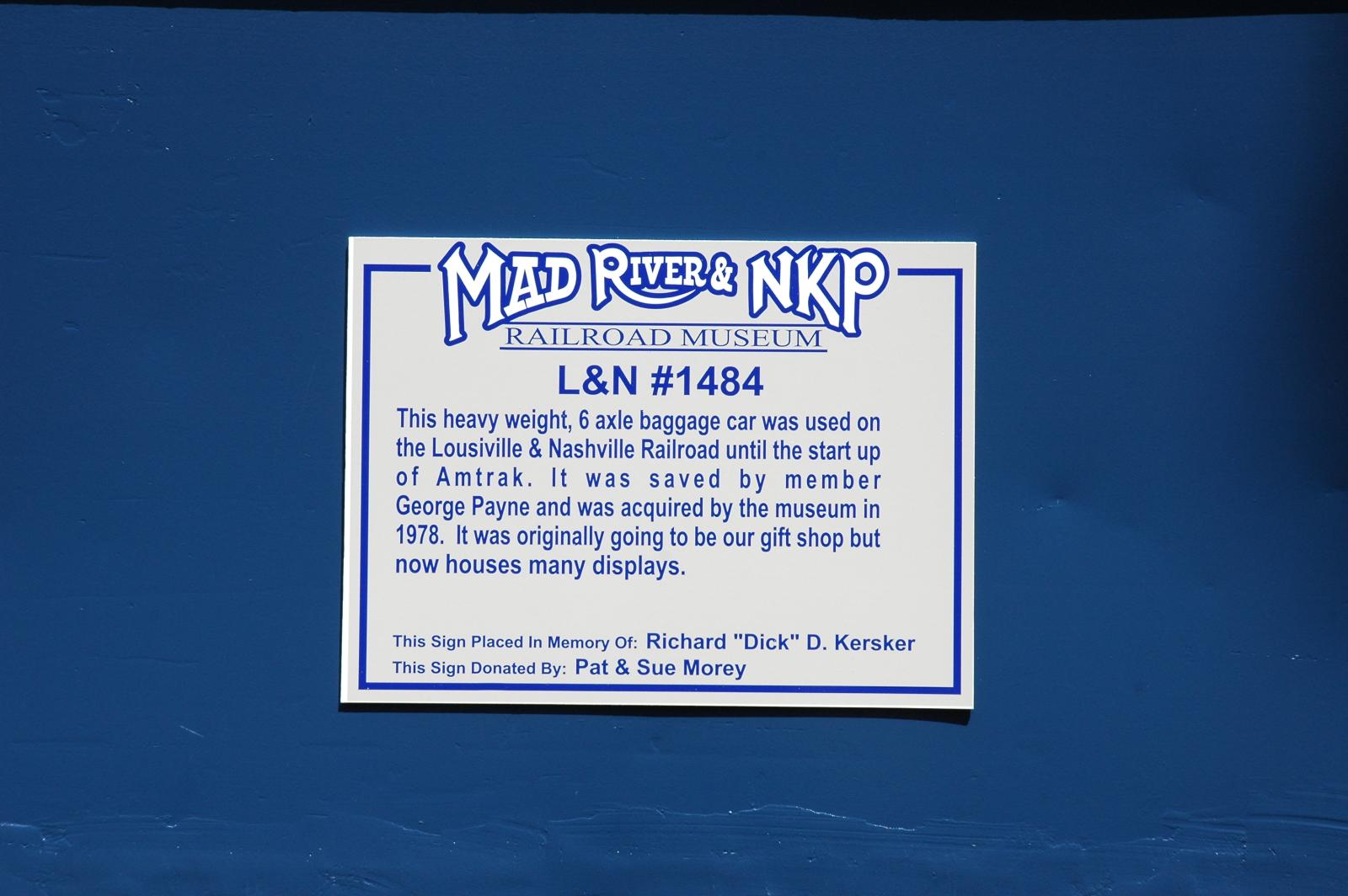The image features a slightly beat-up placard mounted on a solid blue wall. The placard itself is grey with a blue border around its edges. At the very top, "Mad River and NKP" is prominently displayed in white font with a blue border, followed by "Railroad Museum" and "LNN #1484" in blue font. The text explains that the heavyweight six-axle baggage car, originally used on the Louisville and Nashville Railroad until the startup of Amtrak, was saved by member George Payne and acquired by the museum in 1978. Initially intended to be a gift shop, the car now houses numerous displays. The sign is placed in memory of Richard "Dick" DeKersker and was donated by Pat and Sue Morey.